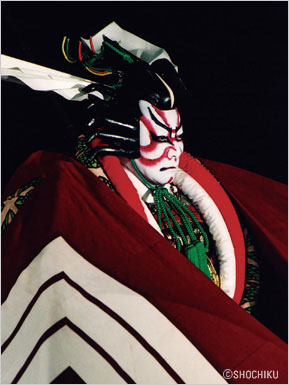The image features a Japanese person prominently displayed against a completely black background. This individual, dressed in traditional Japanese attire, stands slightly in profile, facing to the right. His face is theatrically painted in white with dramatic black stripes across his forehead, and he sports elaborately styled black hair with a striking gold streak forming a widow's peak. Draped over his shoulders is a burgundy flag adorned with white sergeant stripes. Around his neck is a distinctive puffy collar in red and white. His expression is solemn, evoking the image of a historical or ceremonial figure. This detailed and visually arresting portrayal is reminiscent of a character from traditional Japanese theater or a historical cosplay. An inscription, reading "Shou Chiku, copyright," is discreetly placed in the bottom right corner of the picture. The overall color scheme includes accents of pale yellow, green, and blue, adding to the image's rich visual tapestry.